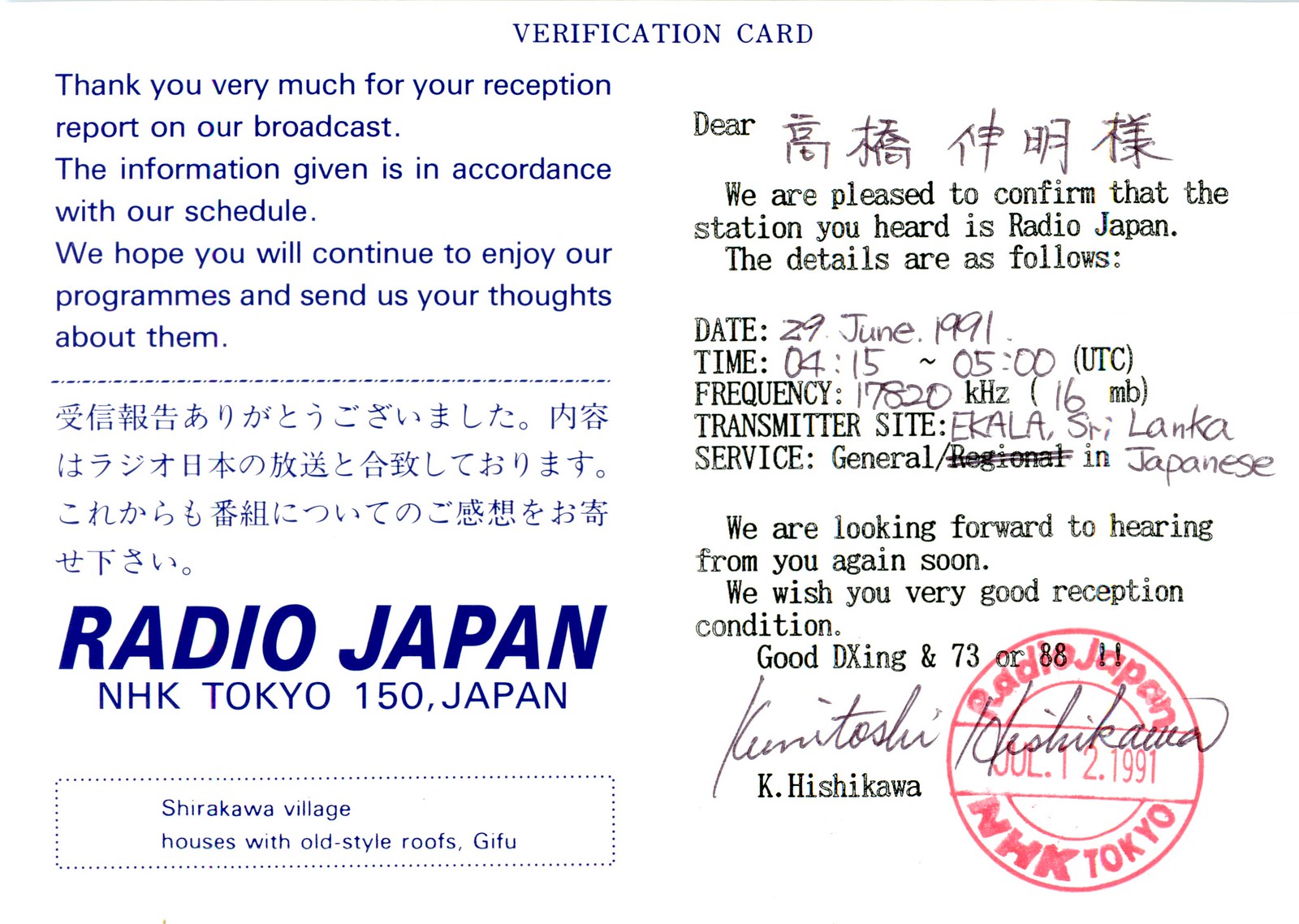The image depicts a postcard-shaped, white background verification card with blue text at the top that reads "VERIFICATION CARD" in capital letters. On the left side, the card contains a thank you note in blue text, which reads, "Thank you very much for your reception report on our broadcast. The information given is in accordance with our schedule. We hope you will continue to enjoy our programs and send us your thoughts about them." This section is followed by four lines of Japanese characters and concludes with "Radio Japan NHK Tokyo 150 Japan." Beneath this, within a border of blue dots, it notes "Shirakawa Village Houses with Old Style Roofs, Gifu."

The right side of the card is divided into several sections of black text, starting with a greeting that includes Japanese characters. It states, "We are pleased to confirm that the station you heard is Radio Japan. The details are as follows," listing the date, time, frequency, and transmitter site. It concludes with a message of looking forward to future reports and wishes for good reception conditions and dining. The section is signed by Kei Hishikawa, with a red circular stamp below that reads "Radio Japan, NHK Tokyo, July 12, 1991."